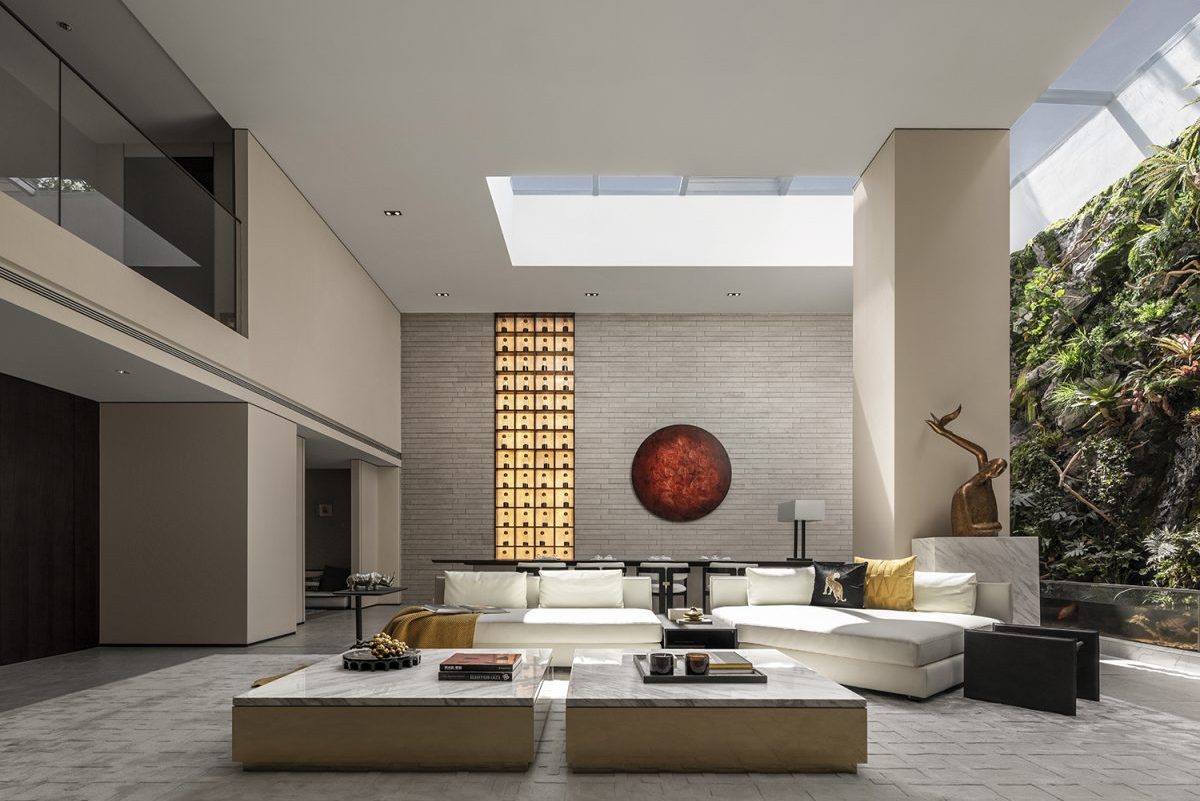This image captures a highly stylized, luxurious, and contemporary living room with a modern, minimalistic design. The room is spacious with high, flat ceilings featuring large skylights in the center and towards the right, allowing ample natural light to flood the space. The floor is made of sleek white marble tile.

Dominating the foreground are two identical rectangular coffee tables with light wood bases and white marble tops, adorned with books, a tray with candles, and various items. Just beyond them, two large, elegant white couches are positioned, offering a comfortable seating area accented by an array of throw pillows. One of the couches slightly curves outward towards the coffee tables, adding a dynamic shape to the arrangement. To the right side of the couches stands a small black end table, and behind them, a black lacquered credenza sits adorned with a lamp that has a black base and a white shade.

The back wall is composed of white brick, featuring a striking round wall decoration with an oriental design in red against a black background. To the left of this graphic, there is a black and gold floor-to-ceiling wall hanging. A tall white stone column, supporting the structure, accentuates the room's height, situated alongside the main skylight.

On the right side, a natural rock wall adorned with various green plants and shrubs brings a touch of nature indoors, complemented by additional skylights above. The left side of the room reveals a two-story layout, with a wide entryway supported by another stone column on the first floor and a spacious white wall with a large horizontal window on the second floor. The overall design masterfully blends contemporary elements with luxurious details, creating an inviting and visually stunning living space.